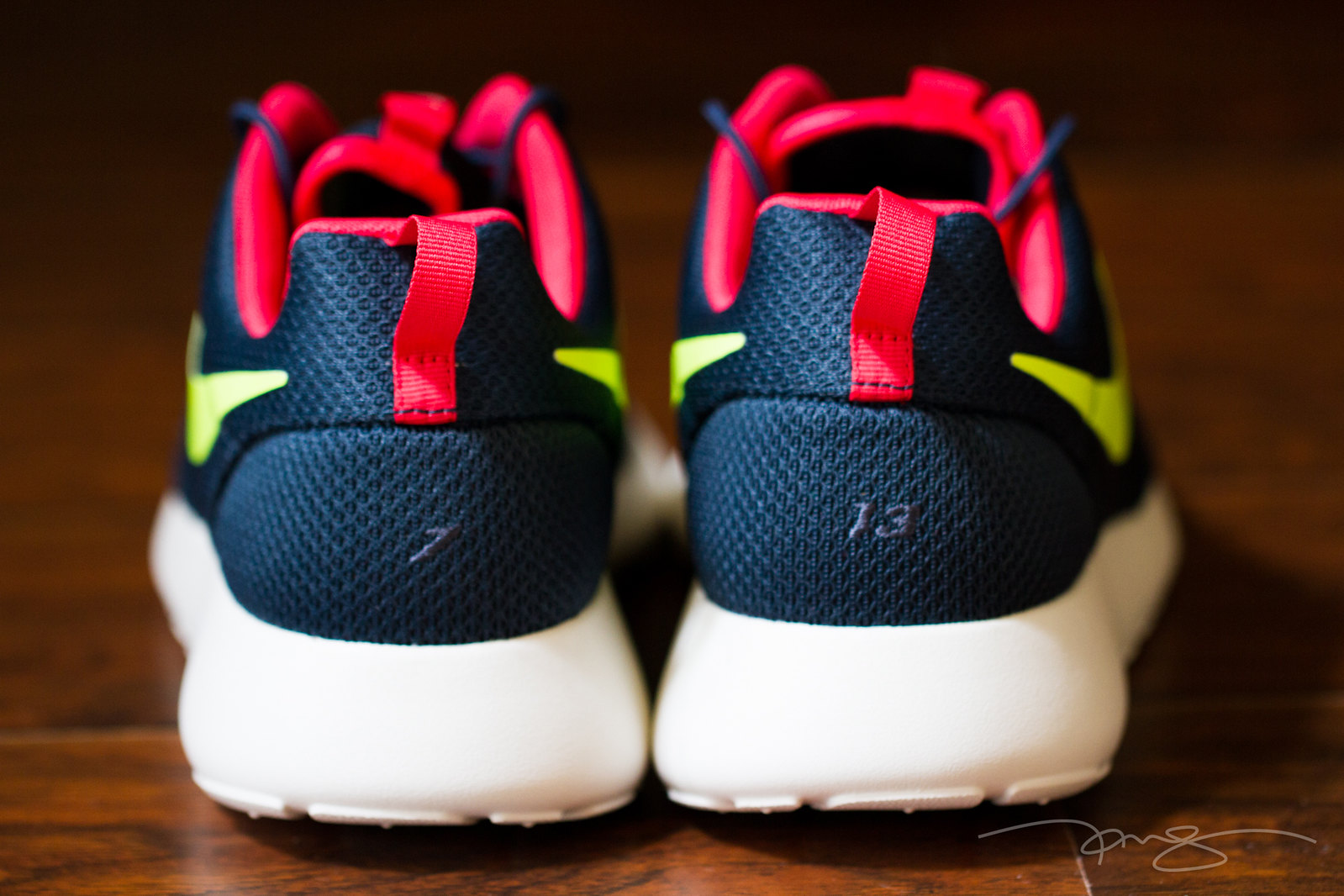This image showcases the back view of a pair of Nike Roche Run tennis shoes positioned on a dark brown hardwood floor. The shoes feature white, chunky, padded soles and a dark blue, breathable material for the main body. A green Nike emblem is visible on the sides. The shoes also have striking red detailing around the mouth and a red pull tab on the back. The left shoe is marked with the number 7, and the right shoe with the number 13. Notably, there is what appears to be a signature in an artsy cursive at the bottom right of the image. The lighting, which casts shadows to the right, suggests that the light source is positioned behind and to the left.